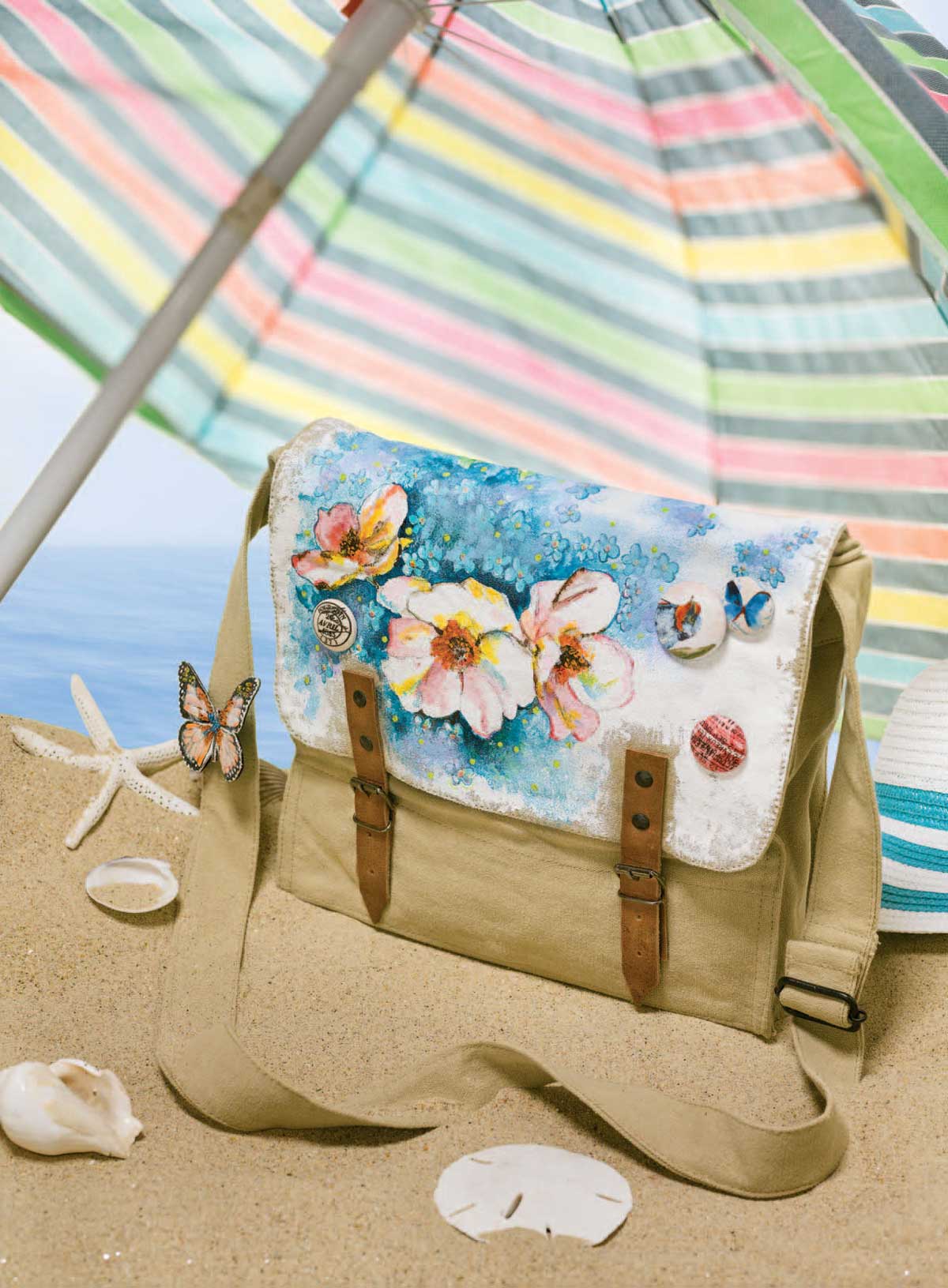A messenger-style bag, primarily brown with a white flap adorned with a floral pattern of blue, yellow, white, and pink flowers, sits on the sandy beach. The bag has a tan strap matching the color of the sand and features several pins, including a distinct butterfly pin on the strap. The bag is positioned centrally, underneath a tilted, multicolored beach umbrella featuring pastel shades separated by black and white lines. The sandy beach beneath it is dotted with various shells and a starfish statue. In the background, the ocean extends to the left, under an extremely foggy sky, creating a serene beach setting.